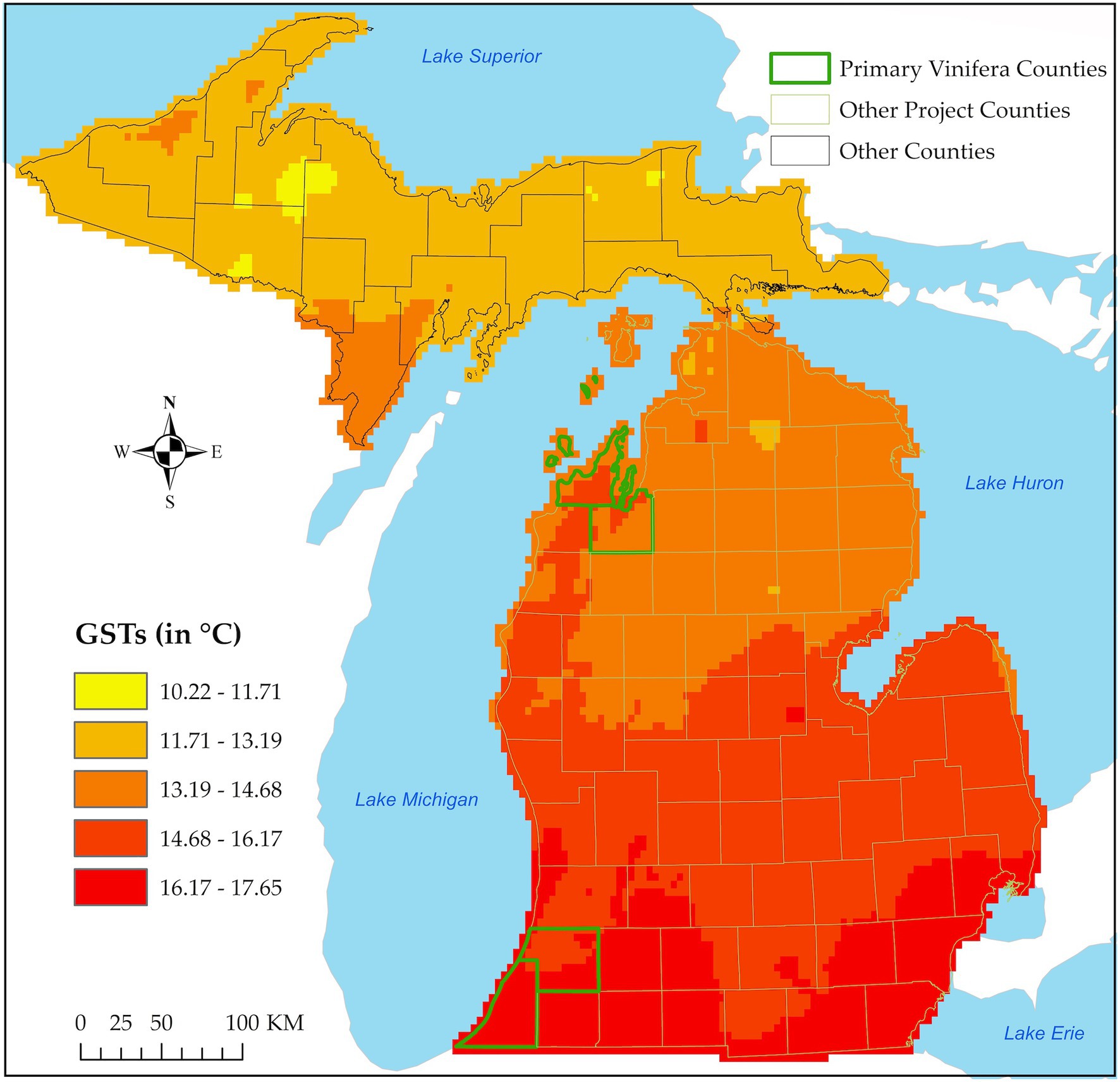This square-format, computer-generated illustration depicts a detailed map highlighting the Great Lakes region, particularly zoomed in on the state of Michigan and its surrounding lakes—Lake Superior, Lake Michigan, Lake Huron, and Lake Erie. The map features a highly detailed heat map indicating temperature variations across different areas, presented in a colour spectrum from yellow to red. The temperature scale, ranging from 10°C to 17.65°C, is shown through a gradient that moves from yellow (cooler areas) to dark red (warmer areas), with specific GST (Growing Season Temperature) ranges marked in degrees Celsius. Key lakes are highlighted in light blue, with Lake Superior positioned at the top, Lake Huron on the right, Lake Erie at the bottom right, and Lake Michigan extending three-quarters up the left of the image. Additional elements on the map include a compass rose indicating cardinal directions, a vertical scale measuring from 0 to 100 kilometers, and colour-coded boxes at the top indicating different counties and projects related to viniculture. The detail in the portrayal of Michigan’s geography and the pixelated depiction underscores the precision of temperature distribution in this region.